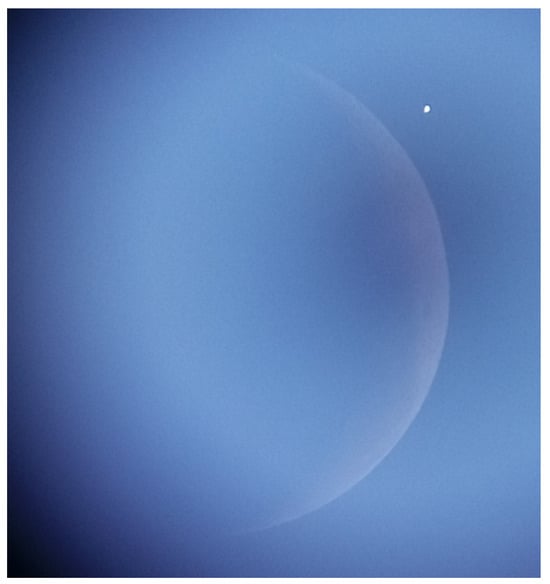The image presents a celestial scene dominated by hues of blue transitioning from a lighter shade on the right to nearly black on the top and bottom corners, lending a vignette effect. A crescent-like celestial body, likely the moon, occupies the right third of the image. This lunar silhouette fades gently into the gradient, with the middle area of the image exhibiting a softer, lighter blue that intensifies to a medium blue towards the far right. The moon's shape is faint and shadowed in the center, with a distinct light spot in the upper right corner of the crescent. A small white speck, possibly another celestial body or an artifact, is visible a few centimeters from the moon, adding a touch of mystique to the overall tranquil and monochromatic celestial tableau.